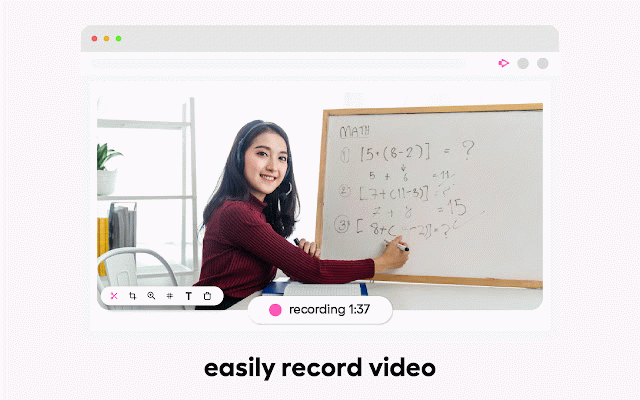The image depicts a blank computer graphic, possibly a screen capture, with a minimal and unfinished interface. The main section is largely empty, suggesting placeholder areas for a heading and text, though no content has been added yet. At the bottom of the screen, there are several small, unclear buttons labeled with various functionalities. In the top left corner, there are three dots colored green, yellow, and red, typically indicating window controls. The top right features an arrow symbol. The overall appearance resembles the interface you might see while waiting for data to load. At the bottom of the screen are several controls: a stop button, a pause button, and a highlighted button with a circular icon on it, with a cursor hovering over it. Additional tools, such as a pen, a rectangle tool, and icons labeled 'stickers' and 'erasers,’ hint that this might be an application related to drawing or editing graphic content.